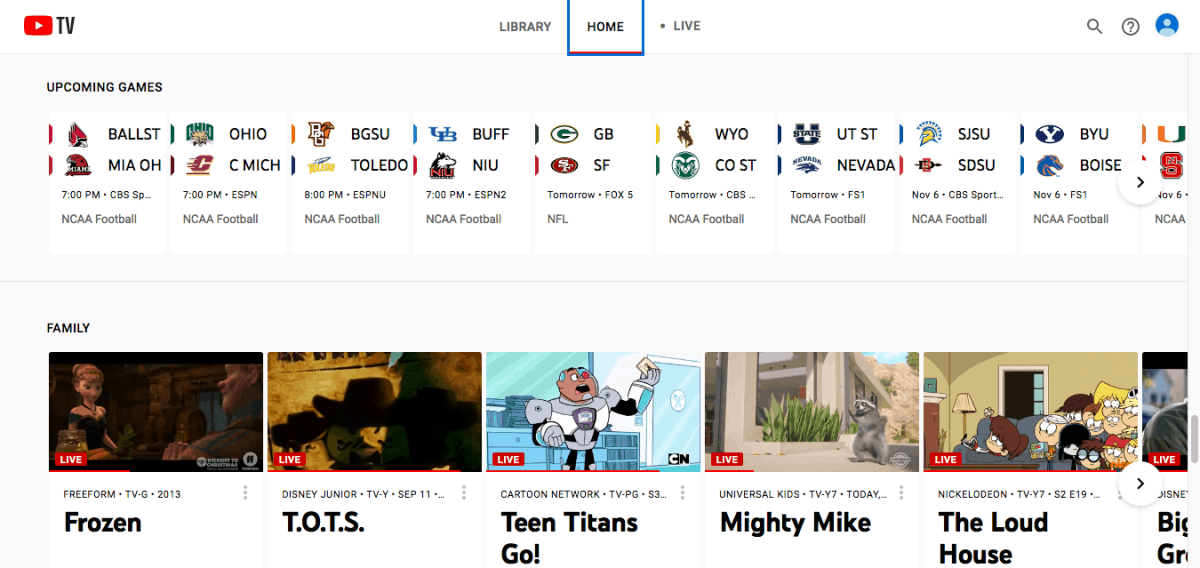The image displays a YouTube TV interface on the "Home" screen. It features a comprehensive guide showcasing various upcoming events and entertainment options. The top section highlights scheduled football games, including Ball State versus Ohio State and the notable Green Bay at San Francisco game set for tomorrow, with specific times listed for both.

Below the sports listings, a "Family" section offers a variety of family-friendly shows. Notable mentions include "Frozen" available on Freeform, "T.O.T.S.," "Teen Titans Go!," "Mighty Mike," and "The Loud House," each accompanied by corresponding thumbnails for easy recognition.

Users have several navigation options: they can scroll down for further listings or use the shuffle function on the right to explore more choices. The interface also allows users to switch between tabs, such as the "Library" for recorded content, "Home," and "Live TV" for current broadcasts.

Overall, the image captures the organized and user-friendly layout of YouTube TV, showcasing its diverse range of programming and intuitive navigation tools.